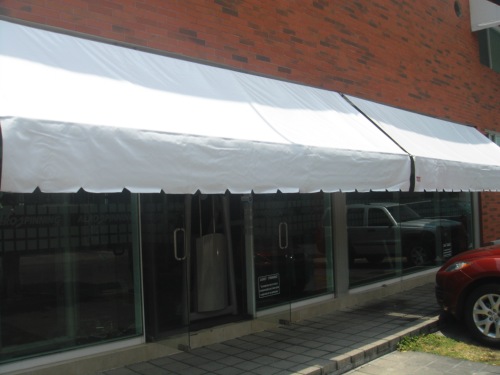This photograph captures the front of a red brick storefront, showcasing a mix of lighter and darker shades of bricks for a textured effect. Above the large row of glass windows and doors, there is a prominent white canopy made from fabric, which extends at a 45-degree angle before hanging down with a distinct triangular cut-out pattern on its edge. The glass doors, which are open, feature sleek metal D-shaped handles. The sidewalk in front of the store is partially shaded by the canopy, and in the bottom right corner of the image, the front of a red vehicle is visible. This includes the left front wheel arch with its black tire and silver rim, as well as part of the headlight, all parked on a patch of green grass.